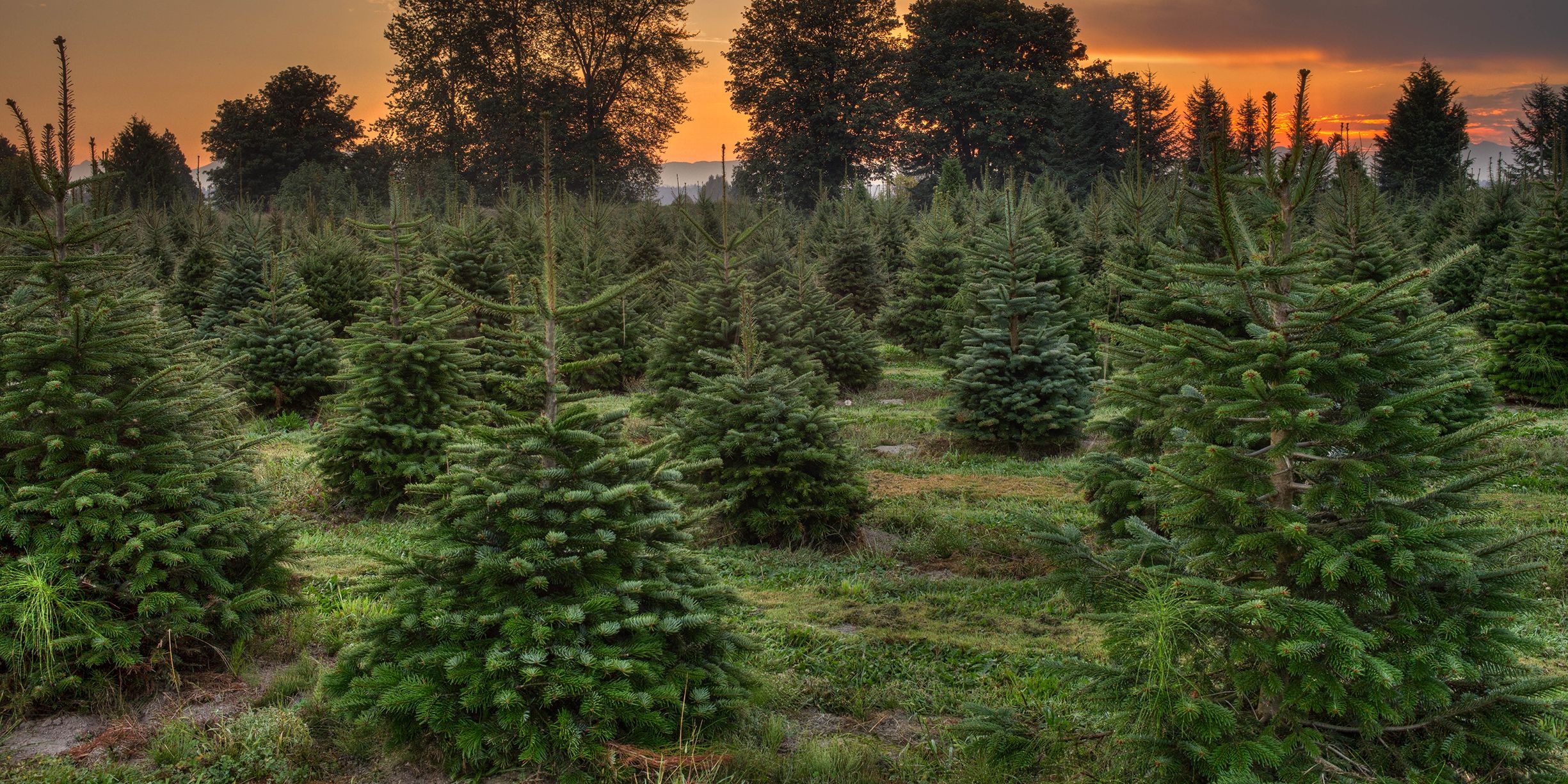This high-resolution photograph taken outdoors captures the serene beauty of a Christmas tree farm at either sunrise or sunset. The scene is dominated by rows of small, green evergreen trees, spread about six feet apart. These trees, not yet fully grown, are nestled in a field of lush, green grass. In the background, there are taller, non-evergreen trees, casting their outlines against the vibrant, orange sky streaked with some clouds. The sky, turning a blend of orange and gray hues, highlights the peacefulness of the setting. Additionally, there are faint hills or a hilly outline visible in the distance, adding to the depth and tranquility of the image. The overall composition, with its rich greens and earthy browns, emphasizes the natural beauty and meticulous arrangement characteristic of a tree farm.